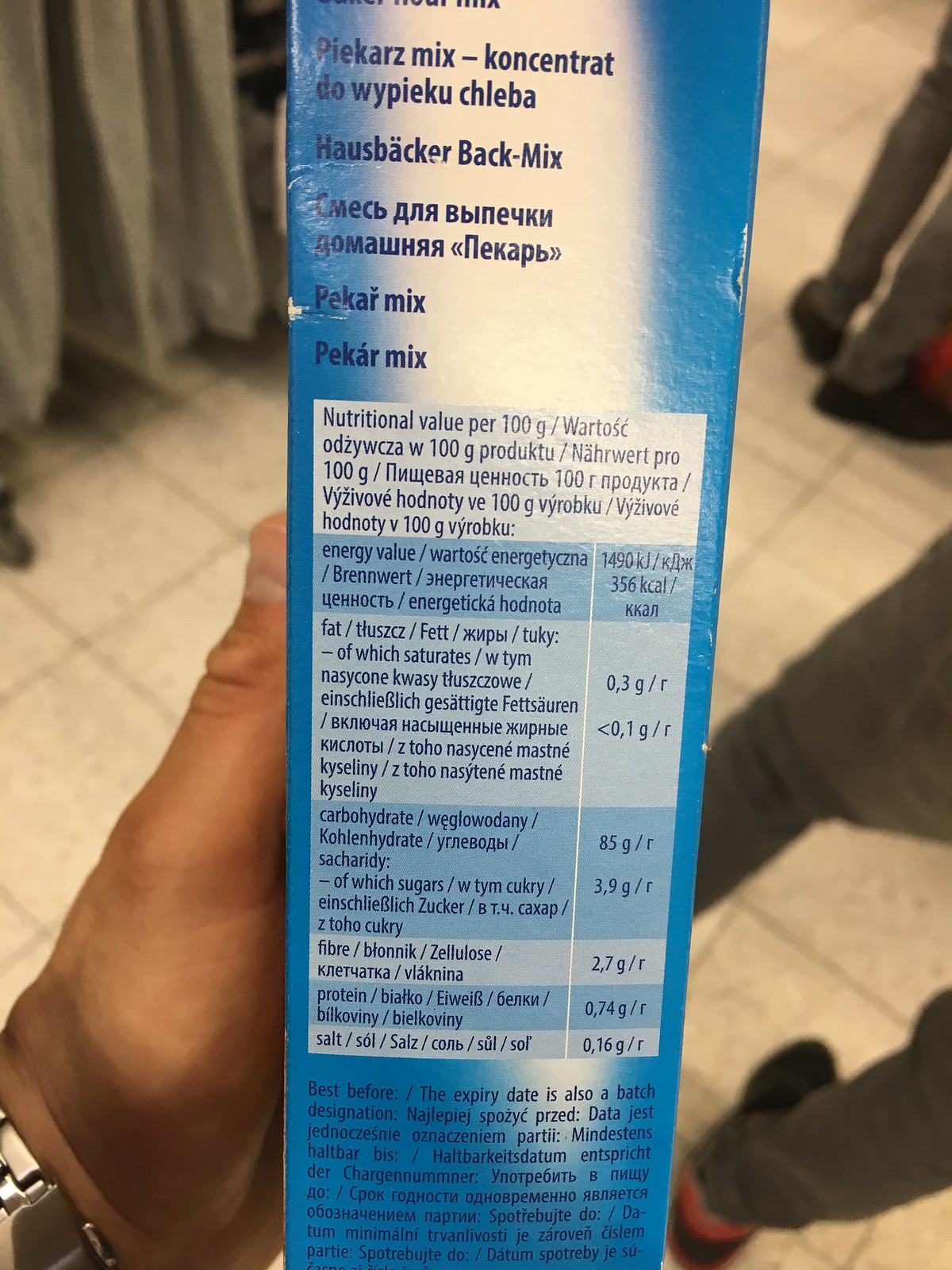This photograph captures a close-up, point-of-view shot of a person holding a blue and white box with nutritional information written in multiple languages, including Russian and German along with some English. The person is in a store with white tiled flooring, holding the box in their left hand, wearing a watch with a silvery wristband. The box prominently features the text "PIEKARZMIXKONCENTRAT DOWYPIEKU CHLEBA HAUSBACKER" at the top in dark blue font. Below this, a white section highlights nutritional values per 100 grams, detailing energy (350 cal, 1490 kJ), fat (0.3 grams), carbohydrates (85 grams, including 3.9 grams of sugar), fiber (2.7 grams), protein (0.74 grams), and salt (0.16 grams). At the bottom, the label mentions a "best before" date alongside a batch designation. In the background of the image, partial views of two other shoppers in grey jeans are visible.